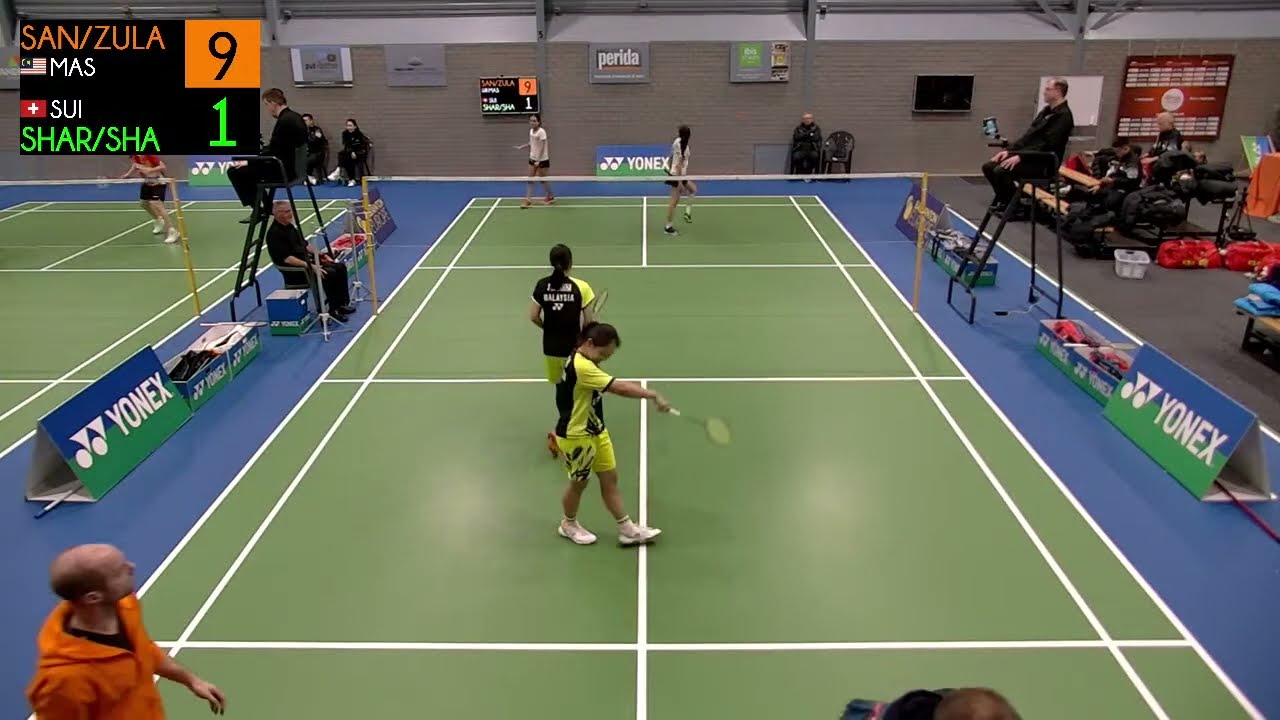The image depicts an indoor doubles match, likely a badminton game, set in a well-lit arena with multiple courts. The primary court has a green floor with white lines and features two players on each side. The players closest to the camera are wearing black and yellow uniforms—black on the back with yellow sleeves and yellow shorts—and they appear to be walking into position rather than engaged in active play. Distinguishing features include elevated nets and players wielding rackets, which suggests a likelihood of badminton, especially with the presence of Yonex advertisements, a known badminton equipment brand.

On the top left of the image, there's a scoreboard displaying the score as "San/Zula: 9" and "Sheriff/Shaw: 1". The team San/Zula appears to have an American flag next to their names and the abbreviation MAS, while Sheriff/Shaw is marked with SUI and a cross, indicating Switzerland. Adding to the scene’s detail, a man in an orange hoodie is visible in the bottom left, and there's a high-standing referee in black attire on the right side of the court, with additional spectators or officials seated behind him. The setting is clear and bright, which enhances the visibility of players and the court layout.